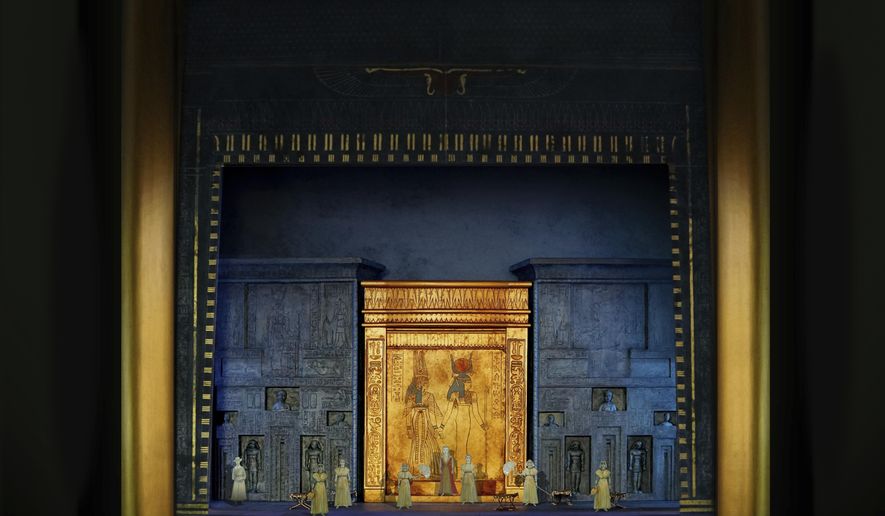The image depicts what appears to be an Egyptian painting set against a solid black colored background, encompassed by a large, ornate gold frame on both the left and right sides. The painting itself exudes a three-dimensional effect, accentuated by the intricate details of three central buildings. The outer two buildings are navy blue with cutaways that reveal figures standing within them, while the middle building gleams with gold and is adorned with Egyptian hieroglyphs and symbols. Prominently featured on this golden central edifice are two Egyptian figures donning blue and red headdresses, distinguished by differing styles. The figure on the left is depicted wearing a long outer garment, whereas the figure on the right sports a sleek, form-fitting dress. Below these structures, the foreground portrays women dressed in long Victorian-era dresses walking along what resembles a street, with some seemingly walking small dogs. The entire scene combines elements of ancient Egyptian aesthetics with what looks like a miniature stage or puppet show, giving an intricate blend of historical and miniature theatrical artistry.